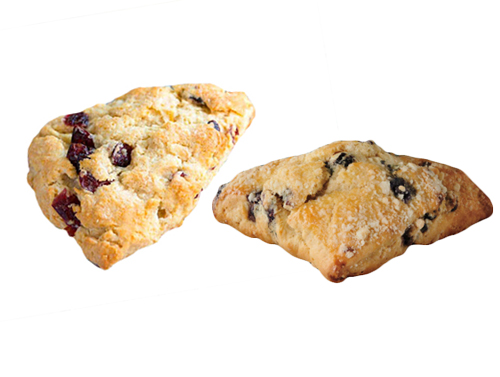This detailed image showcases two delectable scones on a pristine white background. The scone on the left is triangular with a rounded edge, generously filled with what appear to be raspberries, accentuating its appetizing appeal. Its counterpart on the right exhibits a flatter form with a slight peak at the center, adorned with scattered dark blue berries, which may be blueberries or possibly chocolate chips. Both scones share a golden-tan hue, topped with a glistening sprinkle of sugar, lending them an irresistibly sweet and inviting appearance. The scones are positioned side by side, offering diverse perspectives that suggest this image is crafted for an advertisement or menu display, aiming to attract customers with their fresh, baked allure.